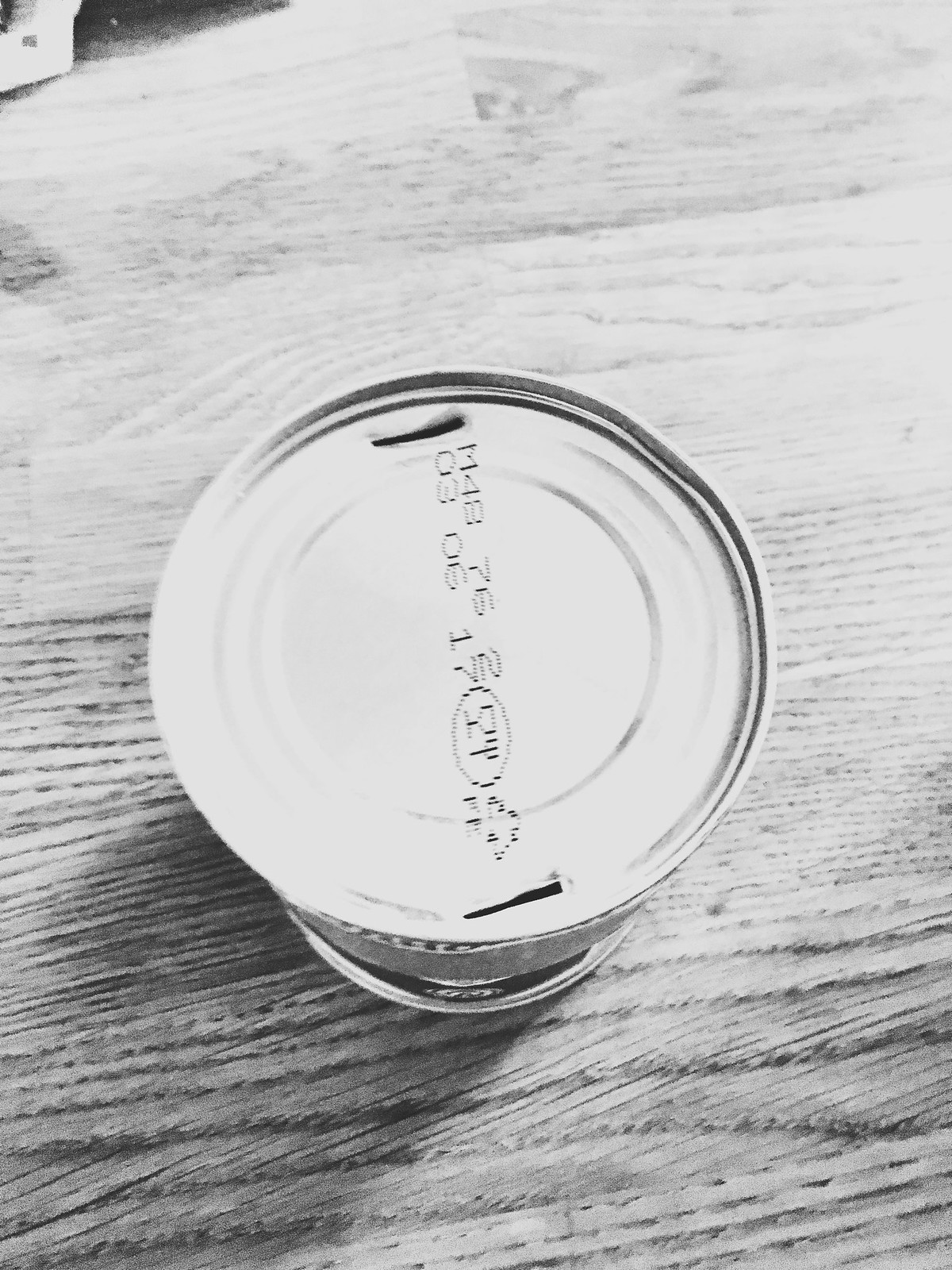A detailed black-and-white photograph captures the top view of a metallic can, likely made of steel, that has been opened using an old-fashioned can opener. This opener leaves distinctive long, slit-like markings on the can's surface; one slit is positioned just near the 12 o'clock mark, while the other slit is located close to the 6 o'clock mark. The can rests on a table with a visible wood grain texture, adding a rustic backdrop to the scene. Between the two slits, there is a section coated in black with alphanumeric characters. These characters are oriented vertically along the top of the can, facing the left side of the image, adding a layer of intrigue to the vintage ambiance captured in the photograph.